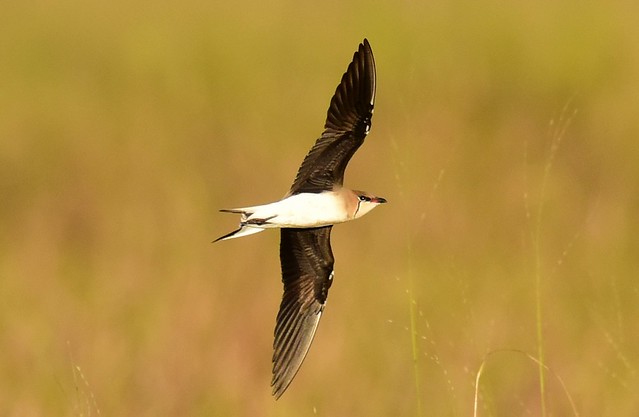This daytime photograph captures a bird soaring mid-air with its wings fully spread, occupying the length of the frame. The bird is shown flying sideways, revealing a detailed side profile. Its prominent features include a white underbelly, a scruffy feathered neck, and dark gray to brown wings. The bird's beak exhibits a touch of orange or red near the tip, while a bit of beige surrounds its small, black eye. Its legs are neatly tucked beneath its body. The background is heavily blurred, characterized by a yellowish-green hue, suggesting a field or weedy area with some tall grasses visible on the right side, enhancing the bird's sharp focus against a muted backdrop.